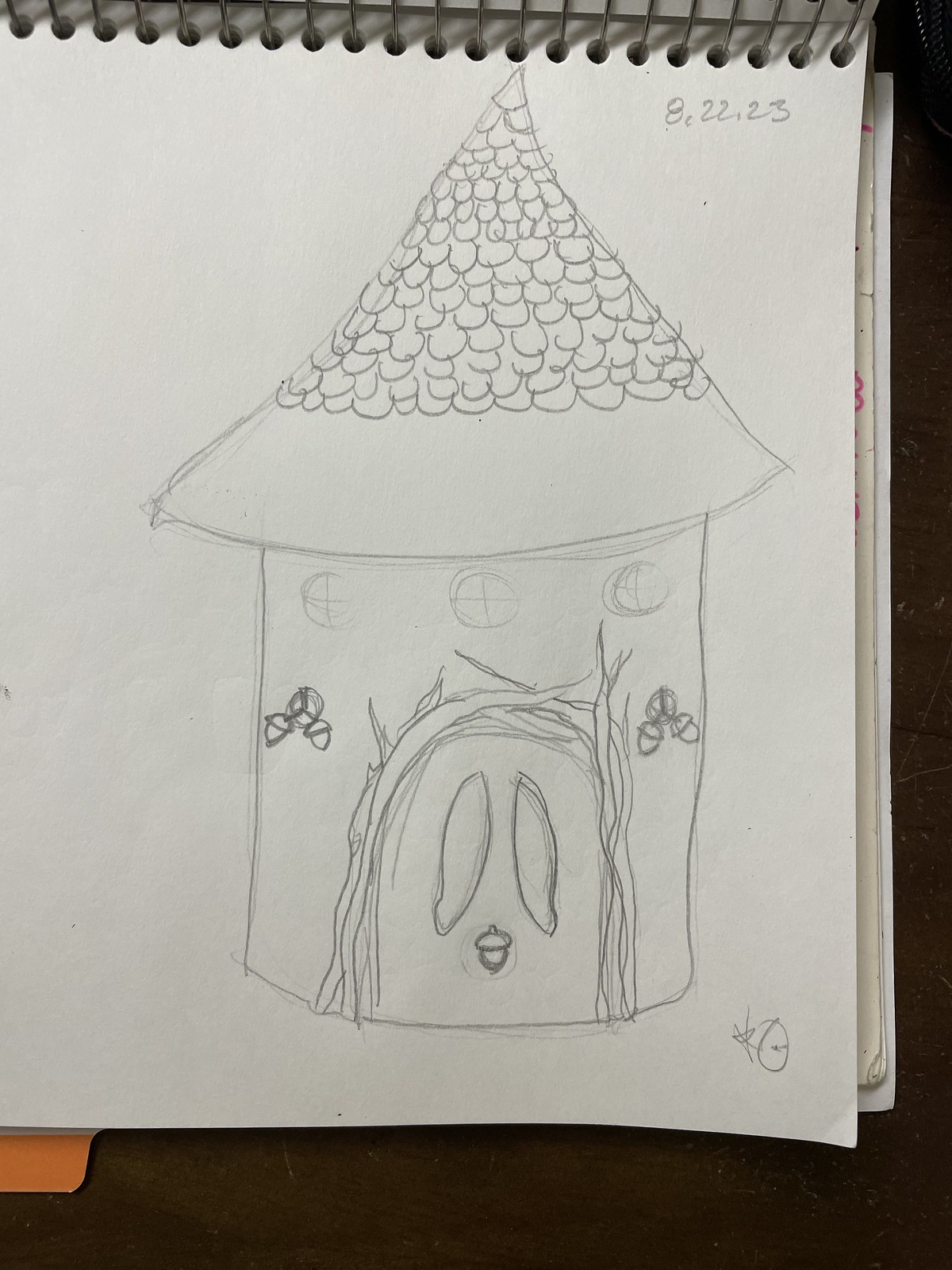The image showcases a detailed pencil drawing on off-white sketch paper from a spiral-bound notebook, with the date 8-22-23 inscribed in the top right corner. The sketch, positioned on a brownish table, depicts an unfinished cylindrical building with a cone-shaped roof, whose tiles cover about two-thirds of the structure. The building features three circular windows each with a cross shape, and a large door adorned with what appear to be roots or vines. The door has two small, spherical windows and is flanked by two hanging acorns on either side, with an additional acorn in the center. The drawing also includes subtle details like a possible signature at the bottom right, and faint lines suggest flowers or acorns beside the door. The inclusion of a bird-like figure with long white eyes and a small beak further enriches the scene.